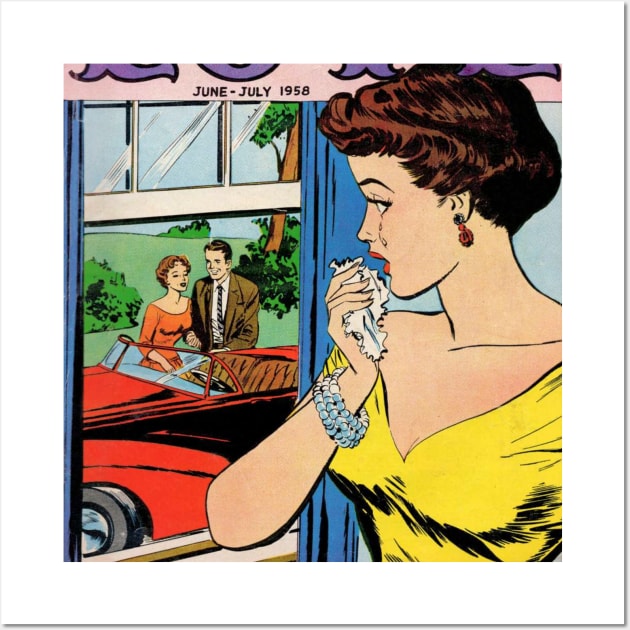The framed square illustration, extracted from a June-July 1958 comic book, portrays a colored cartoon scene through a window with blue curtains. The scene outside the window reveals a bright blue sky, a brown tree trunk, and green bushes. A vivid red convertible with its top down is parked outside. A man with light brown hair, dressed in a light brown jacket, white dress shirt, and black and white striped tie, is seen smiling and opening the car door for a woman with short auburn hair. The woman is wearing an off-the-shoulder orange dress. Inside, next to the open window, stands a woman with short, curled brown hair, her tear-streaked face reflecting her heartbreak. She wears a low-cut yellow dress and a three-banded pearl bracelet. Holding a white handkerchief, she gazes sorrowfully at the man and the other woman, indicating her distress at seeing them together.